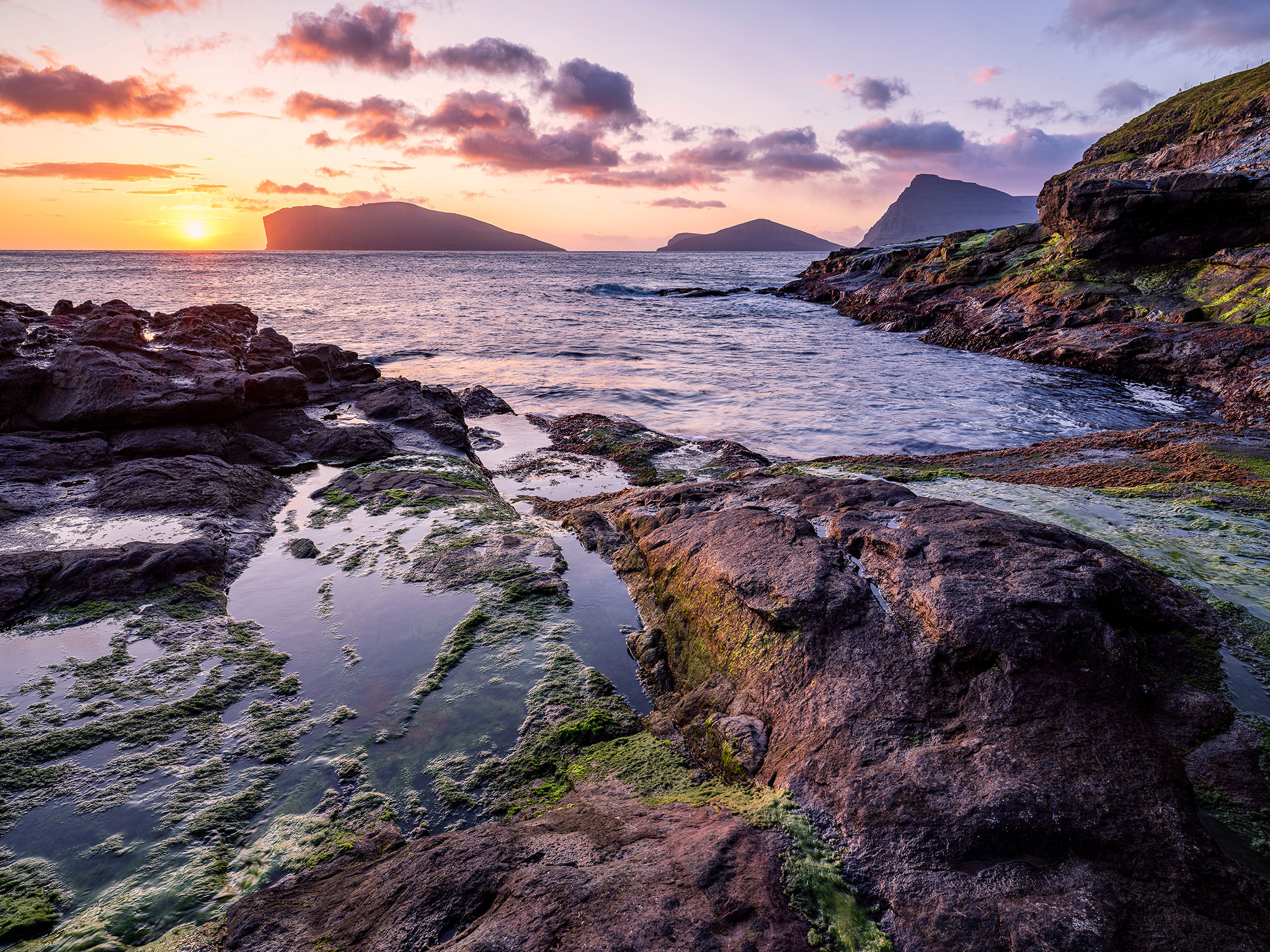This captivating photograph captures a serene sunset scene at an oceanic rocky shoreline with no sandy beach in sight. The foreground features a fascinating tidal pool, formed from receding waves that left behind pockets of water on the rugged, dark gray and brownish rock surface, covered with mossy algae and seaweed. This green growth is prominent and suggests a damp, possibly pungent environment. In the background, the ocean appears rough, contrasting with the stillness of the tidal pools. Far off on the horizon, to the middle and right, large rock formations jut majestically out of the water, resembling steep islets. Dominating the left side of the sky is the setting sun, a radiant golden-yellow orb descending into a colorful canvas of purples, pinks, oranges, and blues. The cloudy sky adds texture to this mesmerizing scene, making this sunset over the ocean a truly peaceful and picturesque sight.